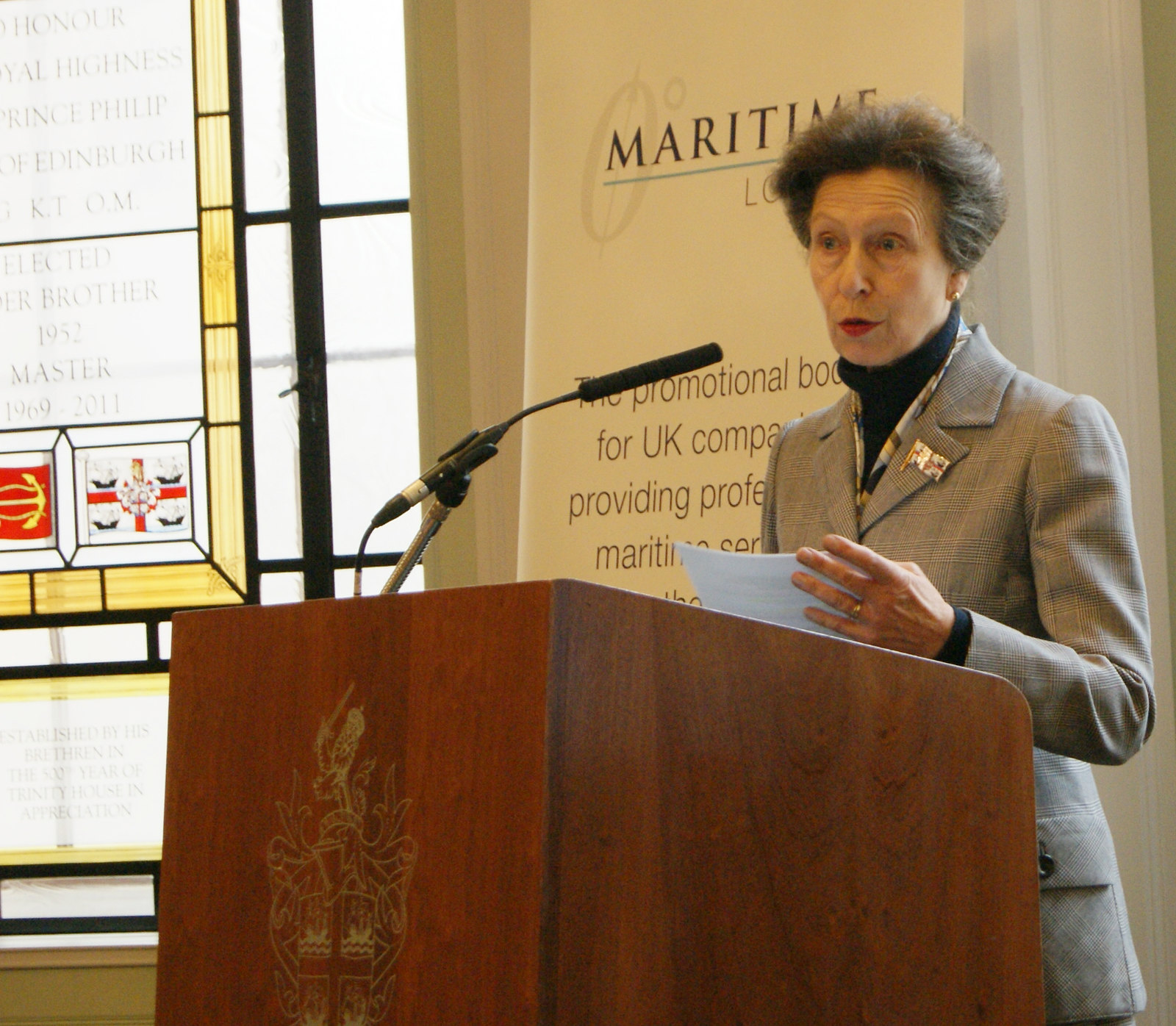In this image, a woman is standing behind a wooden podium with a gold insignia and a thin, black microphone, giving a speech at a formal event. She has short hair, green eyes, and is wearing red lipstick. Dressed in a gray suit with a black turtleneck and a multicolored scarf, she also has a prominent pin on her left lapel. In her hands, she holds a paper while looking out at the audience. The background features a large, mostly clear stained glass window on the left side, adorned with text and insignias, filtering daylight through. There is also a corner of yellow stained glass within a rectangular frame visible. Behind her, a white banner with partial text including words like "maritime" and references to the UK can be seen, likely indicating a promotional event related to maritime activities. The overall setting suggests a serious or significant occasion.